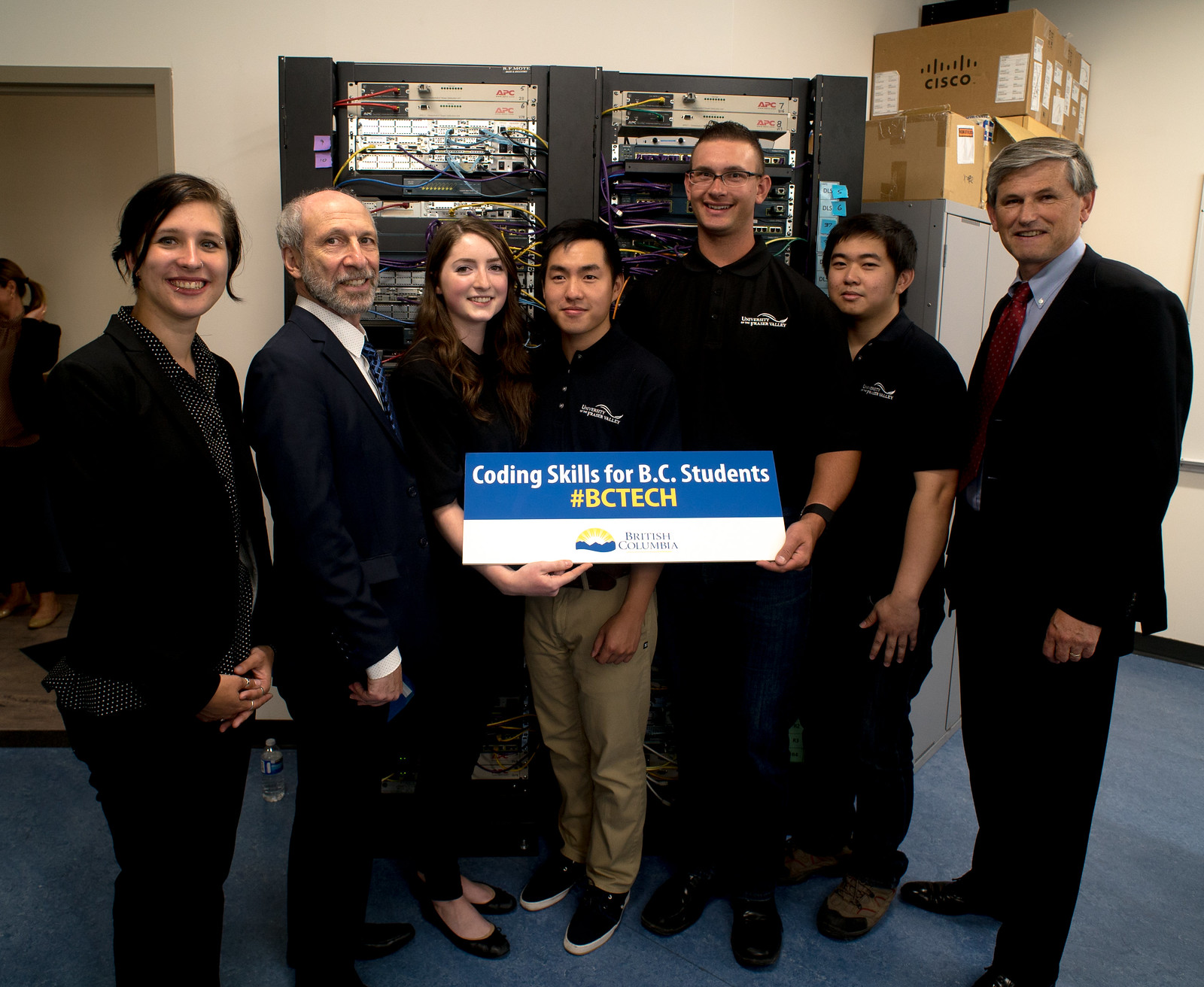This image captures a group of seven individuals standing together in what appears to be a school setting, characterized by a background filled with electronics, including two servers on shelves with visible wires, all set against a beige wall. The scene includes a variety of details, such as a brown door to the left, a filing cabinet crowded with cardboard boxes bearing the Cisco logo on the right, and a blue carpet underfoot.

In the center of the group, they hold a prominently displayed sign that communicates the purpose of their gathering. The sign features a blue stripe with the words "Coding Skills for BC Students" in white lettering and a yellow hashtag "#BCtech," along with the British Columbia logo.

The group consists of five younger individuals, likely students, and two older gentlemen, likely the instructors. From left to right, we have:

1. A woman dressed in black pants, a suit jacket, and a polka dot shirt.
2. An older, balding man in a dark suit with a white shirt and blue tie, who also sports a beard.
3. A woman with long brown hair, similarly dressed entirely in black.
4. A man in a black polo shirt and khaki pants.
5. Another man in a black polo shirt and dark pants.
6. Yet another man wearing the same black polo shirt and dark pants.
7. An older man in a suit with gray hair, a blue shirt, and a red tie, standing on the far right.

The detail and arrangement suggest a formal yet collaborative atmosphere, emphasizing the teaching and learning of coding skills in British Columbia.